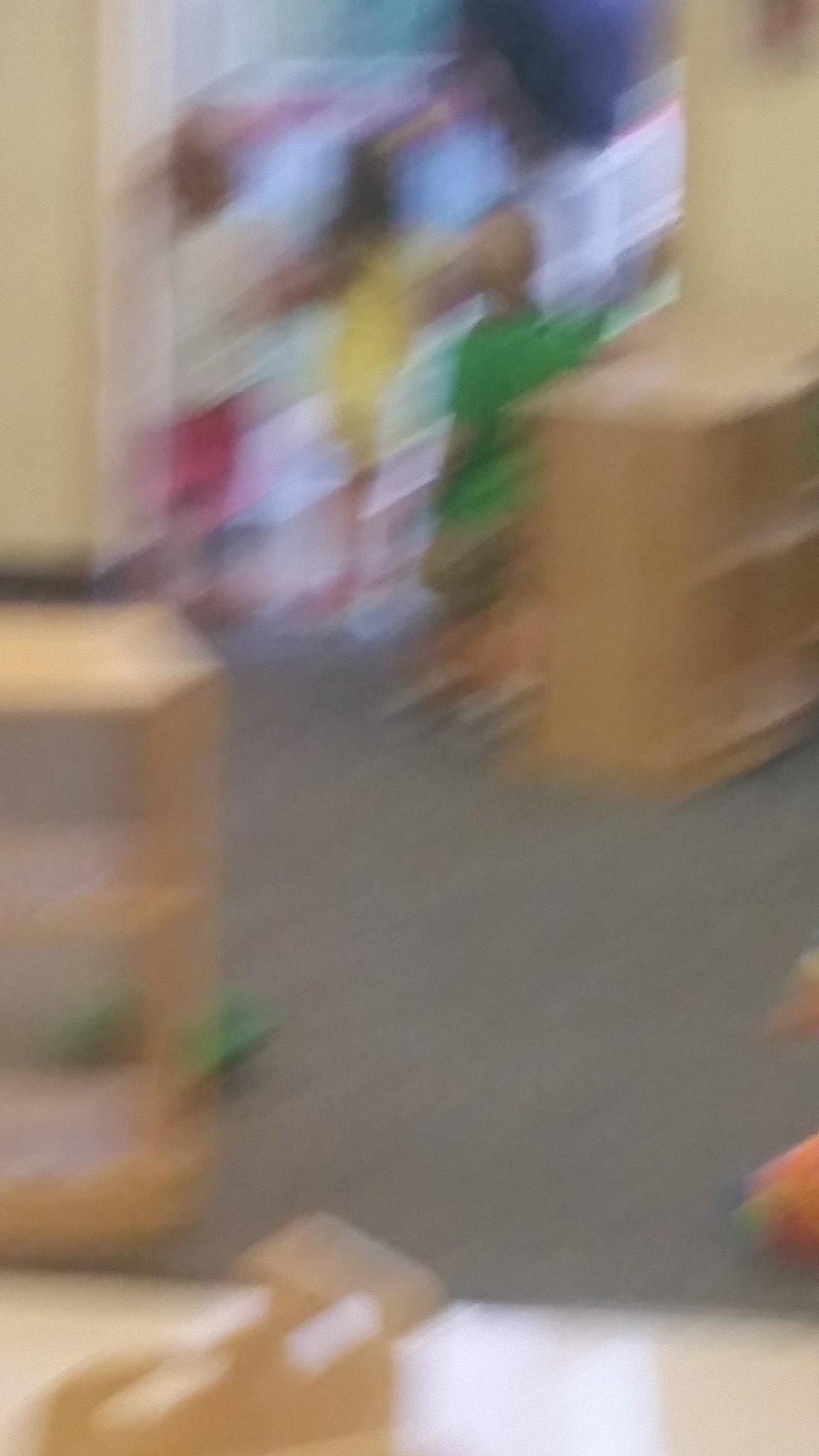This photograph, taken indoors, appears to capture a lively scene from either a daycare or a children's library, although it is very blurry. In the foreground, there are two short shelves visible, possibly filled with books or toys. In the background, an adult is interacting with three children. One child is wearing a white shirt paired with pink or red shorts, another is dressed in a yellow outfit, and the third is in a green outfit. The adult, who is partially visible, is wearing white pants and boots. Despite the image's blurriness, the joyful atmosphere of a children's space is apparent.